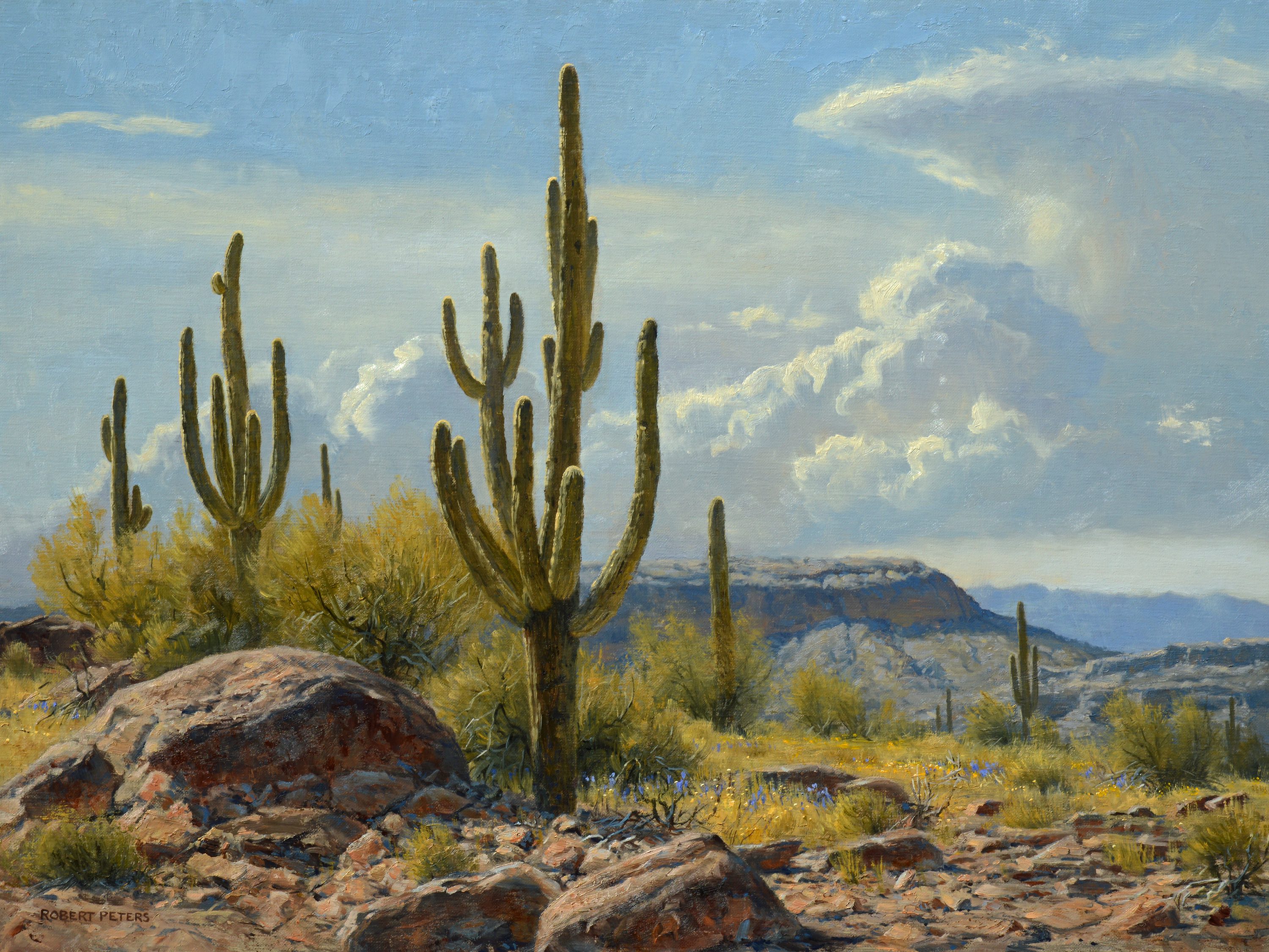The image depicts a semi-realistic, southwestern desert landscape rendered in a painting style that tries to emulate naturalistic scenery. Stretching across the canvas, the sky is a pale blue adorned with stylized, detailed clouds resembling cotton balls. Prominent in the foreground are numerous tall, many-branched cacti, some with as many as fourteen branches. These cacti share the terrain with red, craggy rocks and occasional green bushes and tumbleweeds, hinting at a dry, rugged environment. The background features gray and tan mountains, possibly the Grand Canyon, extending above the horizon and casting shadows that add depth to the scene. Adding a personal touch, the name Robert Peters is signed in the bottom left-hand corner, suggesting the artist of this meticulous painting.